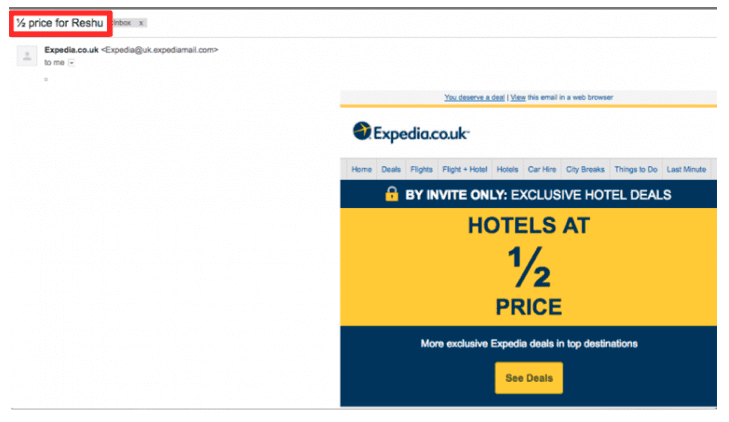This page is for Expedia UK, featuring a streamlined layout that guides the user effectively. The design starts with a prominent black line running horizontally across the top of the page. In the upper left-hand corner, there is a heavily outlined red rectangle with a white interior. Inside this box, bold lettering reads "Half Price," followed by the numerical figures associated with the offer, though these numbers are unspecified for the feature named Reschew. The red rectangle overlaps an adjacent grey box.

A secondary light grey line runs horizontally below the red rectangle. Directly beneath this line is a white square icon that features a person symbol along with the text "expedia.co.uk" in bold, black letters. An arrow points left from this icon, indicating a pathway to a website.

In the lower section, further to the right, there is a prominent square that boldly proclaims, "We Deserve a Deal," followed by a vertical line. The text that follows mentions something about an email in a web browser, but the specifics are unclear.

Below this section, there is a gold line, followed by the recognizable Expedia logo with the accompanying text "expedia.co.uk." The header concludes with navigation options, totaling 11 tabs, starting from "Home," "Deals," "Flights," and "Flight and Hotel," among others. The design is both visually structured and informative, encapsulating everything from promotional offers to navigation options effectively.